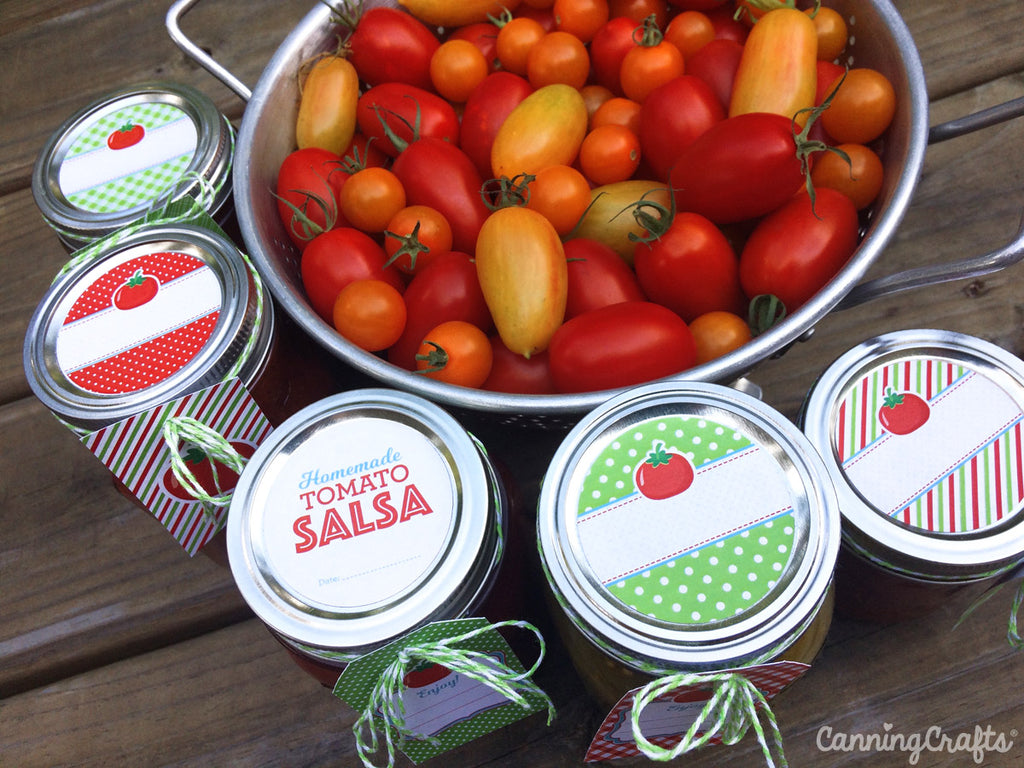The image depicts an overhead view of a rustic brown wooden table, conveying the essence of a cozy, homey atmosphere. Dominating the upper portion is a large, round metal bowl with silver handles, brimming with a vibrant mix of tomatoes in a spectrum of colors—yellow, orange, red, and various shades in between, each adorned with green stems.

Below the bowl and more prominently displayed are five mason jars filled with homemade salsa, each sealed with uniquely decorated lids. The lids feature various designs, including green and red polka dots, stripes, and checkered patterns, often with a central image of a red tomato with green leaves. One jar in particular stands out with a label that reads "Homemade Tomato Salsa" in bold red and green letters, capturing the essence of its contents. 

Some jars also differentiate themselves with charming ribbons tied around them, serving as additional labels. The attention to detail and the careful presentation make it evident that these salsas were crafted with care using fresh, homegrown tomatoes.

In the bottom right corner, elegantly written in cursive white text, the words "Canning Crafts" are displayed, underscored by a registered trademark symbol, adding a professional touch to the artisan presentation of the homemade goods. The entire scene is bathed in natural light, enhancing the vivid colors and textures, and emphasizing the clarity and quality of the image.